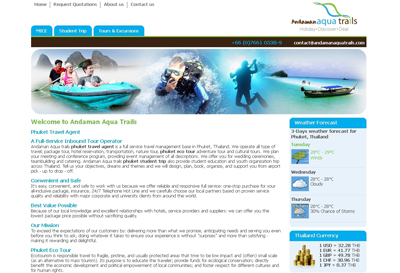At the top left of the image, there are navigation tabs labeled "Home," "About Us," and "Contact Us." To the right, the heading "Awkward Trails" is prominently displayed. Below this heading, the image features a series of visuals:

1. A picture of three people in a canoe with giant rocks in the background.
2. An image capturing a scuba diver both underwater and partially above water.
3. A boat resting on the shore of a beach.

Beneath these images, the text "Welcome to Awkward Trails" is written, followed by several paragraphs of text in blue font. The layout consists of multiple paragraphs each featuring blue text. 

On the right side of the image, there's a section with a blue border at the top, followed by black text. This section includes:
- A picture of a tree.
- A picture of clouds.
- A picture of the sun partially obscured by a cloud.
Below these images, there's another blue border featuring what appears to be a stack of gold coins and some blurred, nonsensical words next to it.